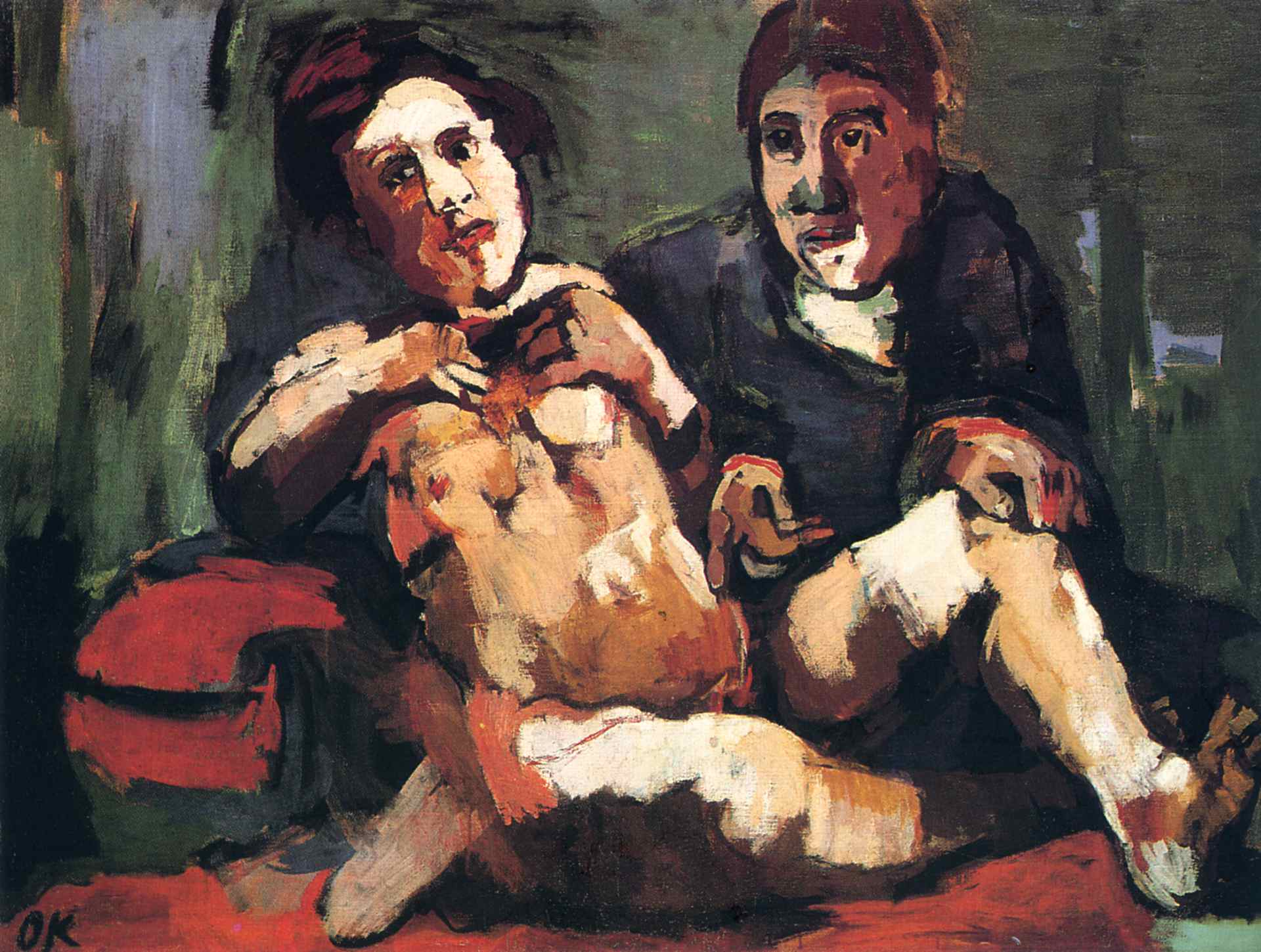The painting is a large, borderless square canvas, featuring two central figures against a background composed of blended brush strokes in green, blue, and black hues, making the setting ambiguous. On the left, there is a person who could be a woman or possibly a man; this figure appears naked, with short brown hair and a slightly open mouth, gazing off to the left. The body shows different shades of brown, particularly around the belly and breast areas, suggesting possible pregnancy. The individual has an arm that might be leaning on an armrest, and their legs extend out in front, displaying patches of white and brown, potentially indicating a bandage on the left knee. 

To the right sits a man with short brown hair, clad in a dark blue shirt. He is seated slightly behind the foreground figure, also looking to the left, with his hand resting on the other's knee. The ground on which they sit is painted in red, which, combined with other details, like a potential chair's armrest, suggests they might be on a red couch or table. Additional colors, such as baby blue in the top left corner and light green to the side, add complexity to the background. The signature "OK" is visible in black paint at the bottom left of the painting. The overall style features a multitude of shapes, adding to the painting's dynamic nature and suggesting themes of birth or human connection.